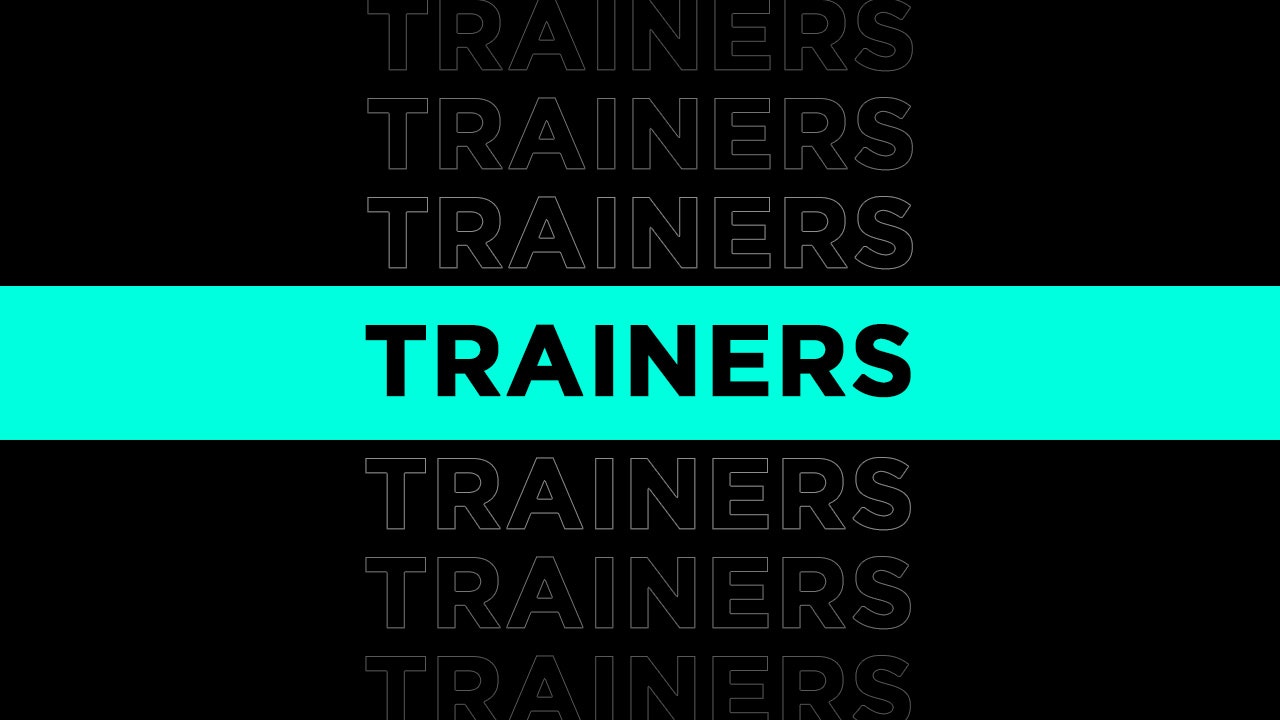The image features a simple, graphic design with a black background. Central to the composition is the word "TRAINERS" repeated vertically down the middle, seven times in total. These letters are outlined in a thin gray or off-white, forming a visually repetitive pattern. In the center of the image is a horizontal teal or mint green stripe, creating a striking contrast against the black background. Within this teal strip, the word "TRAINERS" appears again, this time in solid black letters matching the background above and below it. The overall layout resembles that of a presentation slide or digital banner, with a clean, rectangular format and a modern, minimalistic style.